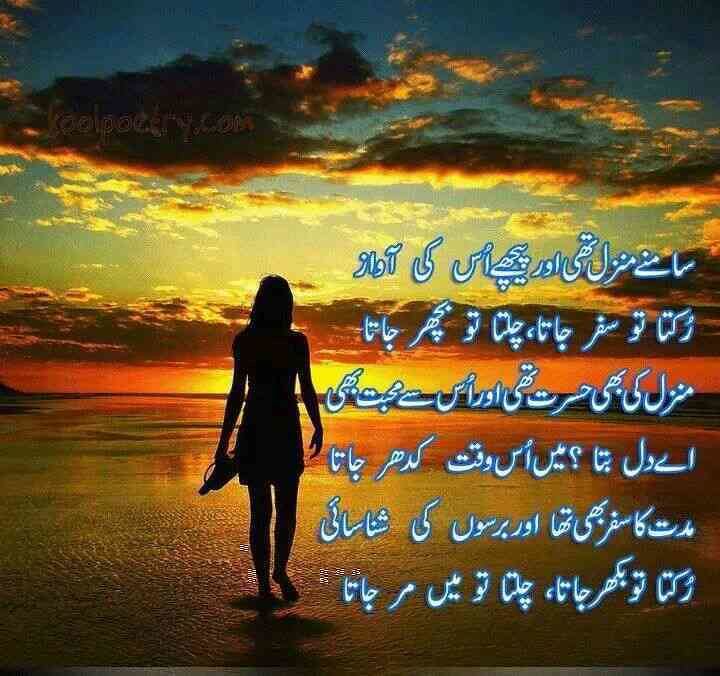The image is a square digital artwork featuring a quote overlay. Just left of center, a silhouette of a woman in a short skirt and potentially a t-shirt or t-shirt dress walks away on a sandy surface that mirrors the colors of a sunset, extending into a shallow, transparent body of water. The sunset paints the water and shore in hues of orange. The woman holds flip-flops in her left hand, her right toe extended up slightly. Above her, the sky transitions from deep turquoise at the top to yellow and blue in the middle, becoming redder and darker toward the horizon. Two distinct cloud layers are present: thick, blocky clouds with edges of burnt orange and bright yellow covering the sun, and more stringy clouds on the left. In the upper left corner, a faint watermark reads "coolpoetry.com". To the right of the woman, there are six lines of text in a language that resembles Arabic or Farsi, outlined in light blue. The image quality is low, giving it a slightly indistinct appearance.